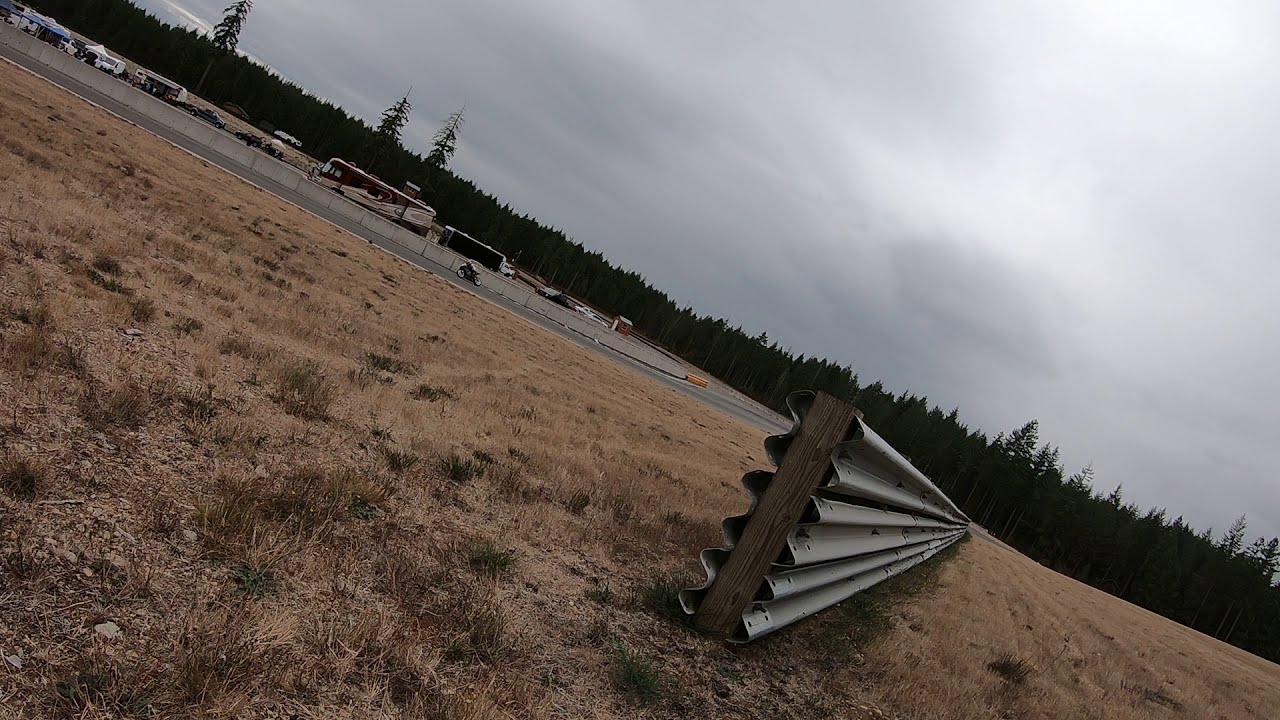This outdoor photograph captures a landscape dominated by dead and brown grass, indicative of an arid or seasonal environment. A metal guardrail mounted on wooden posts stands out in the foreground, to the right side of the image, adding a hint of infrastructure amidst natural elements. Scattered rocks punctuate the grassy terrain. In the midground, a road stretches across the scene, occupied by a motorcycle. Beyond the road, there is a parking lot on the left side, filled with large vehicles including buses, trucks, and RVs, adding a sense of travel and transit to the setting. The distance is enveloped by a dense array of tall evergreen trees, silhouetted against an overcast sky. The sky itself is gray and hazy, with thick clouds blocking most of the sunlight, casting a muted light over the entire scene. The overall composition suggests a rest stop or a roadside area, blending elements of nature and human activity.